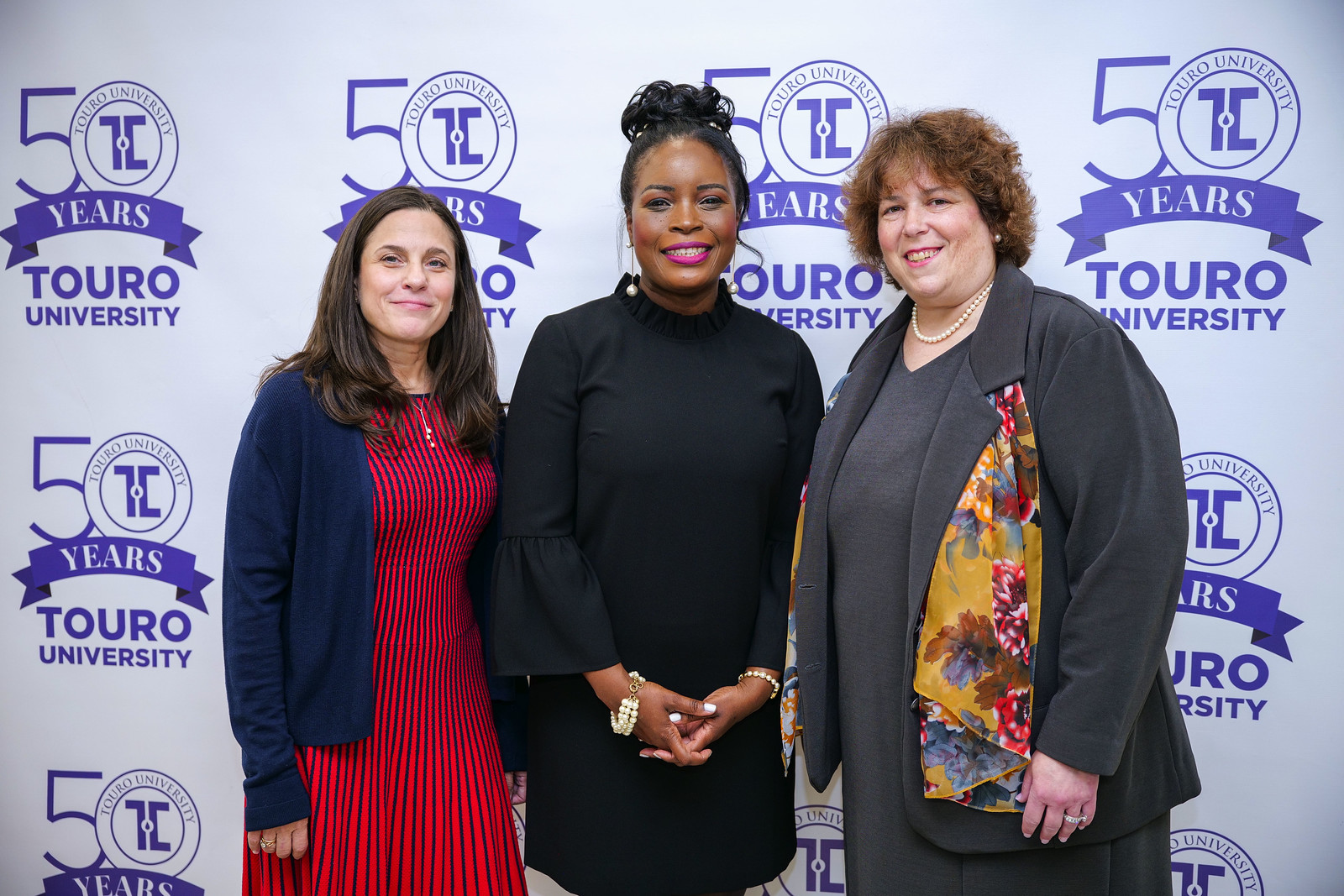The image captures three women standing in front of a light blue backdrop that features repeated text and logos commemorating "50 years" of Touro University. From left to right, the woman on the left is a shorter white woman with shoulder-length brown hair and a light complexion. She is adorned in a blue shawl over a red dress with vertical black stripes, and accessorized with a necklace. The middle woman has dark brown skin and her black hair is styled in an updo. She dons a black dress with long open sleeves, pink lipstick, and wears bracelets and possibly a watch on her wrists. The woman on the right is larger in stature, with short curly brown hair. She is dressed in a gray jacket over a gray dress, accented by a multicolored floral scarf and a pearl necklace. All three women are smiling brightly at the camera.